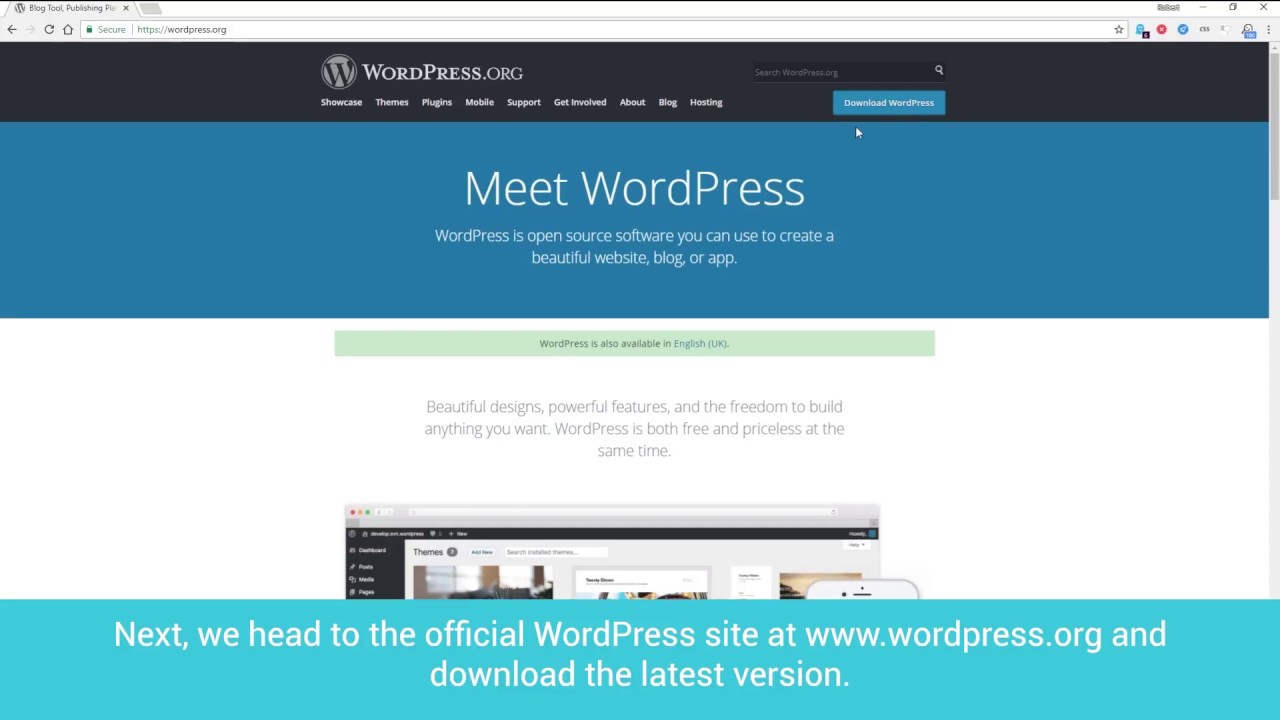Screenshot of the Official WordPress Website

At first glance, this is a detailed screenshot of a web browser window displaying the official WordPress website, wordpress.org. The top navigation bar includes options such as Showcase, Themes, Plugins, Mobile, Support, Get Involved, About, Blog, and Hosting, with a distinctive blue button labeled "Download WordPress" prominently positioned nearby.

Beneath this navigation bar is a large header within a blue rectangle featuring white text that reads, "Meet WordPress. WordPress is open source software you can use to create a beautiful website, blog, or app." Following this introduction, the next section features a white background with a green rectangle that highlights, "WordPress is also available in English (UK)." In this section, the text "(UK)" is presented in blue font.

Below this section, the website emphasizes the versatility of WordPress with the text, "Beautiful designs, powerful features, and the freedom to build anything you want. WordPress is both free and priceless at the same time." An accompanying image illustrates how WordPress may appear on a computer screen.

To explore or download the latest version of WordPress, visitors are directed to the official site at www.wordpress.org.